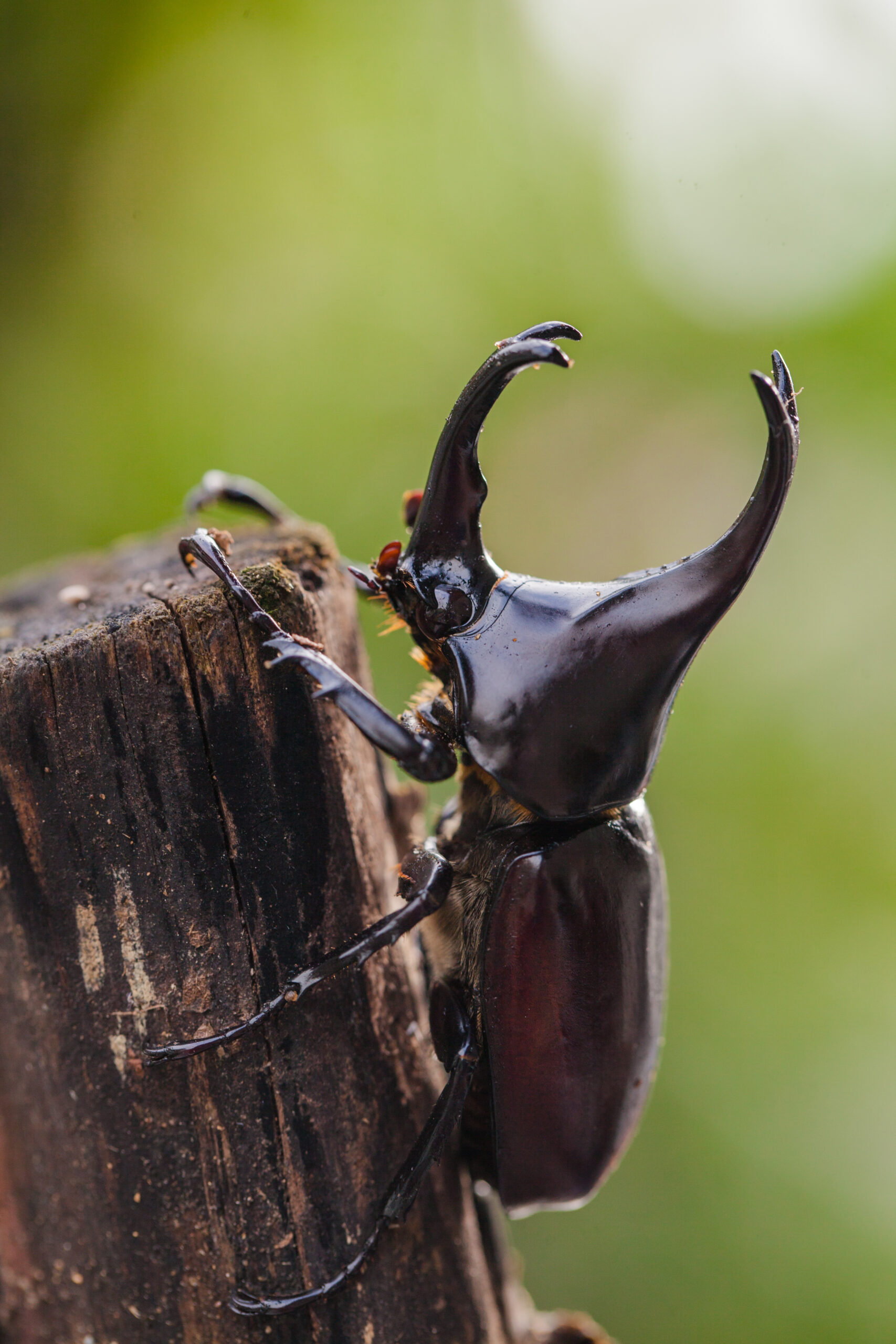The close-up color image captures a unique horned beetle clinging to the weathered end of a brown, rotting piece of wood, possibly a stump or small tree branch. The beetle is displayed in profile, facing to the left, with its shiny black body featuring a slight brown tint on the lower half. Distinctively, the beetle boasts two horn-like prongs on its head; one protrudes upward in front of the eyes, and another extends from above, both interconnected towards the back. The insect features six legs, each with finger-like appendages, with three legs visible in the image as it vertically grasps the wood with its front claws. The background is a blurred green, indicative of an outdoor natural setting. Overall, the beetle appears to be about five inches long and the piece of wood shows signs of weathering and rot.